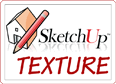In this grayscale image, the background is composed of vertically arranged, grayish planks of wood with visible, darker stripes at the top and bottom edges of each plank. These planks, resembling thick tiles, are connected in two aligned horizontal rows, each featuring five planks. Small, circular screws are depicted in the corners of these planks, adding a touch of detail to the surface. At the center of the image, a watermark showcases a simple sketch of a small house with a door and a window, alongside a pencil positioned diagonally as if resting against the house’s roof. Encircling this central design, the text "SketchUpTextureClub.com" appears repeatedly, forming an oval with additional occurrences of the same text on either side of the circle, creating a cohesive, branded focal point.